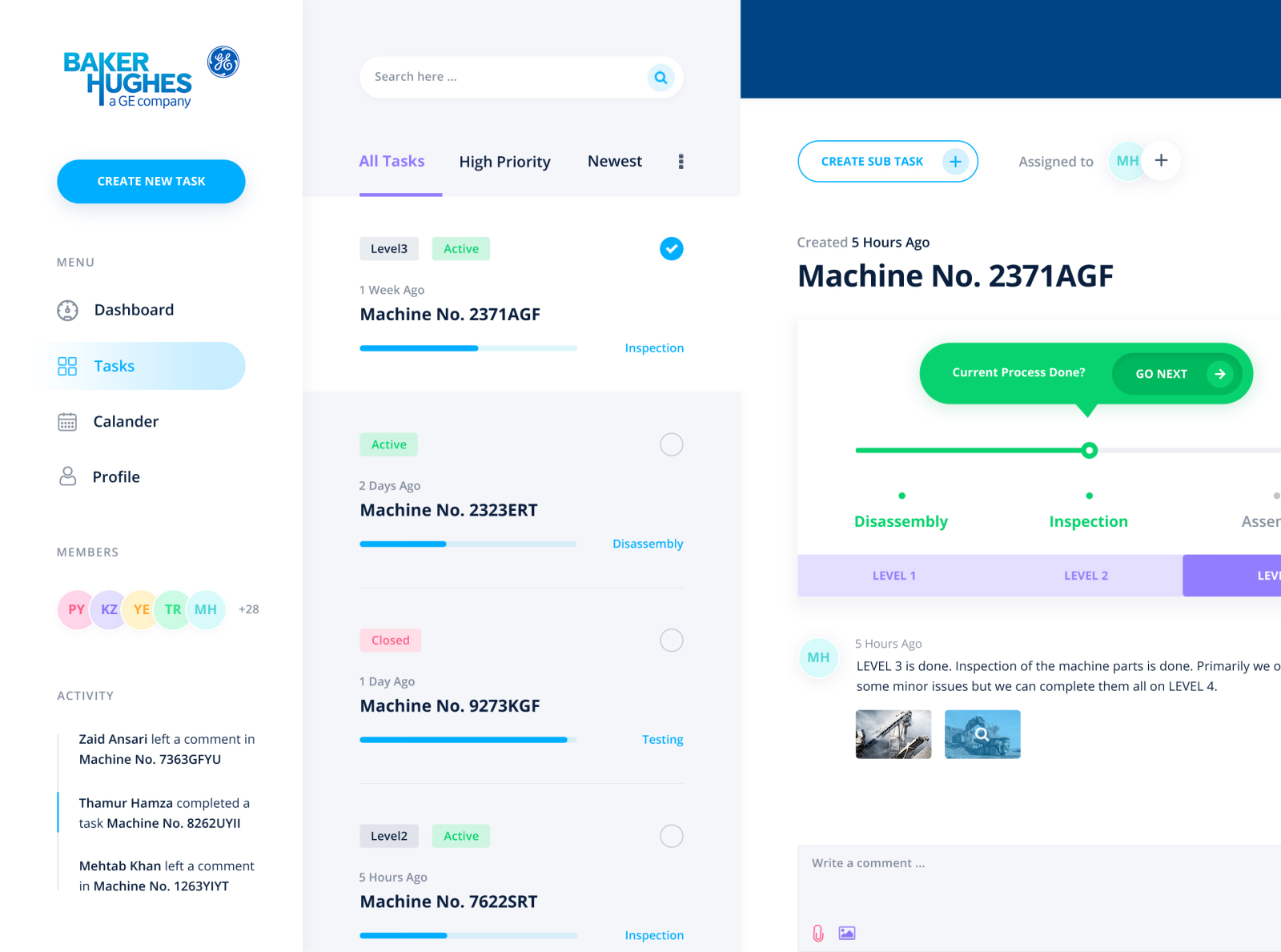The image shows a detailed interface of an application designed for workers at General Electric (GE), specifically for task management. On the left side, the screen displays a section titled "Baker Hughes" with an option to create a new task. Below this, there's a menu button that opens to essential functionalities like "Dashboard," "Tasks" (currently selected), "Calendar," and "Profile." This section also indicates "28+ members" and showcases a list of recent activities, including comments associated with specific machine numbers.

The middle column features a search bar alongside filters for "All Tasks," "High Priority," and "Newest." Additionally, it reveals the task level, status (active), and progress details. Four machines are listed, each with different stages: one for inspection, one for disassembly, one for testing, and another for inspection.

To the right, Machine #2371AGF is highlighted, with a current task of inspection. The usual task sequence is inspection, disassembly, inspection, and assembly, but it appears there is a function to override this progression. Below, it specifies that level three is completed and includes images depicting the steps taken to achieve this completion.